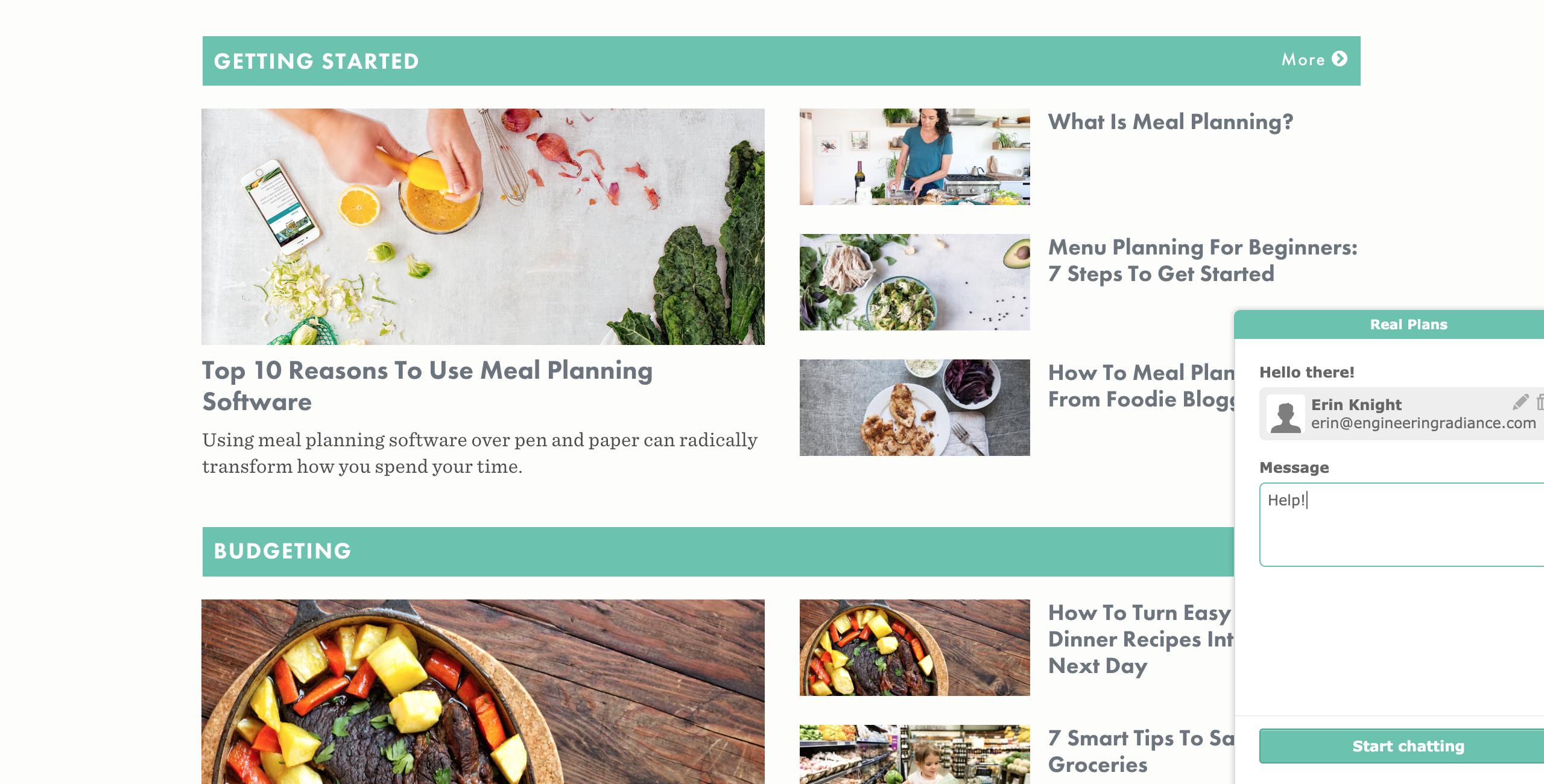The image shows a website layout featuring a green banner with blue hues at the top, displaying the text "Getting Started" in white. Positioned to the right, a clickable element labeled "More" with a capital 'M' and accompanied by a white circle containing a right-pointing arrow is visible.

Beneath the banner is a visually engaging graphic. On the left side of this graphic, a close-up of a woman's hand squeezing a lemon over a bowl is depicted. Surrounding the bowl are various cooking items: a whisk, a halved lemon, a smartphone, some greens, and additional bowls. The accompanying text reads "10 Top Reasons to Use Meal Planning Software."

Adjacent to this scene, three distinct image panels are arranged vertically. Each panel contains a title and corresponding image. The first panel is titled "What is Meal Planning?", the second "Menu Planning for Beginners: Seven Steps to Get Started," and the third "How to Meal Plan."

An overlaying pop-up partially obscures the screen, displaying the text “Meal Plans. Hello there. This is Erin Knight at erinatengineeringgradients.com.”

Below, another banner, labeled "Budgeting," features a partial image of food. However, the text next to it is also obscured by another pop-up, which prevents further details from being discerned.